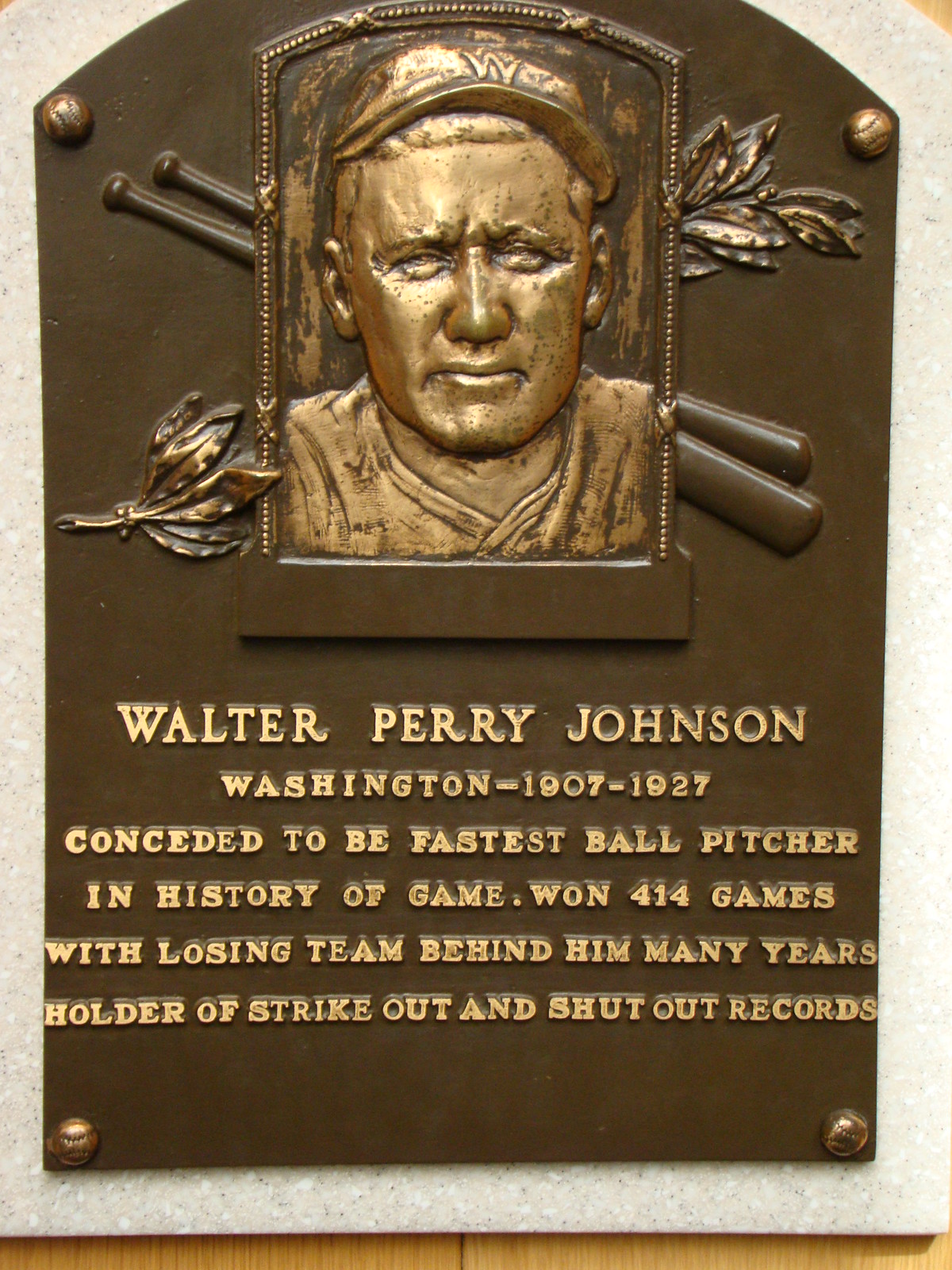This photograph captures a detailed plaque reminiscent of those found at Cooperstown. The plaque is predominantly brown with intricate gold embossing, featuring a prominent image at the top. This image is not an actual photograph but an embossed rendering of the honoree, Walter Perry Johnson. Behind his stern, forward-gazing portrait are two crossed baseball bats, adding context to his celebrated career. The text below his likeness is rendered in bold, capital letters and reads:

Walter Perry Johnson  
He played for Washington from 1907 to 1927.  
Conceded to be the fastest ball pitcher in the history of the game.  
Won 414 games with a losing team behind him many times.  
Holder of strikeout and shutout records.

Additional details include the appearance of plants to the sides of the plaque, enhancing its aesthetic. The overall craftsmanship and informative content of the plaque vividly commemorate Johnson's remarkable achievements and enduring legacy in baseball history.